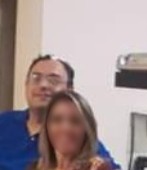The image depicts a low-resolution, thumbnail-sized photo of two individuals in a brightly lit room with white walls. The woman, positioned in the foreground, has long, brown hair with blonde highlights cascading down both sides of her head. Her face is blurred, suggesting a need for anonymity, but it can be inferred that she is smiling. She appears to be wearing a brown coat or a dark long shirt, but the exact details are indistinguishable due to the image's small size. Behind her stands a man, slightly higher in the frame, with a friendly smile. He wears glasses, a blue collared or polo shirt, and his short brown hair is thinning or receding. His face, though visible, is indistinct because of the image's poor resolution. To the right of the image, there are some ambiguous metal objects, one of which is partially visible and rectangular with a dark spot, while another resembles a miniature metal sofa on a black rectangle. Additionally, a gray area on the left side of the image could indicate a doorway or an indented section of the wall.